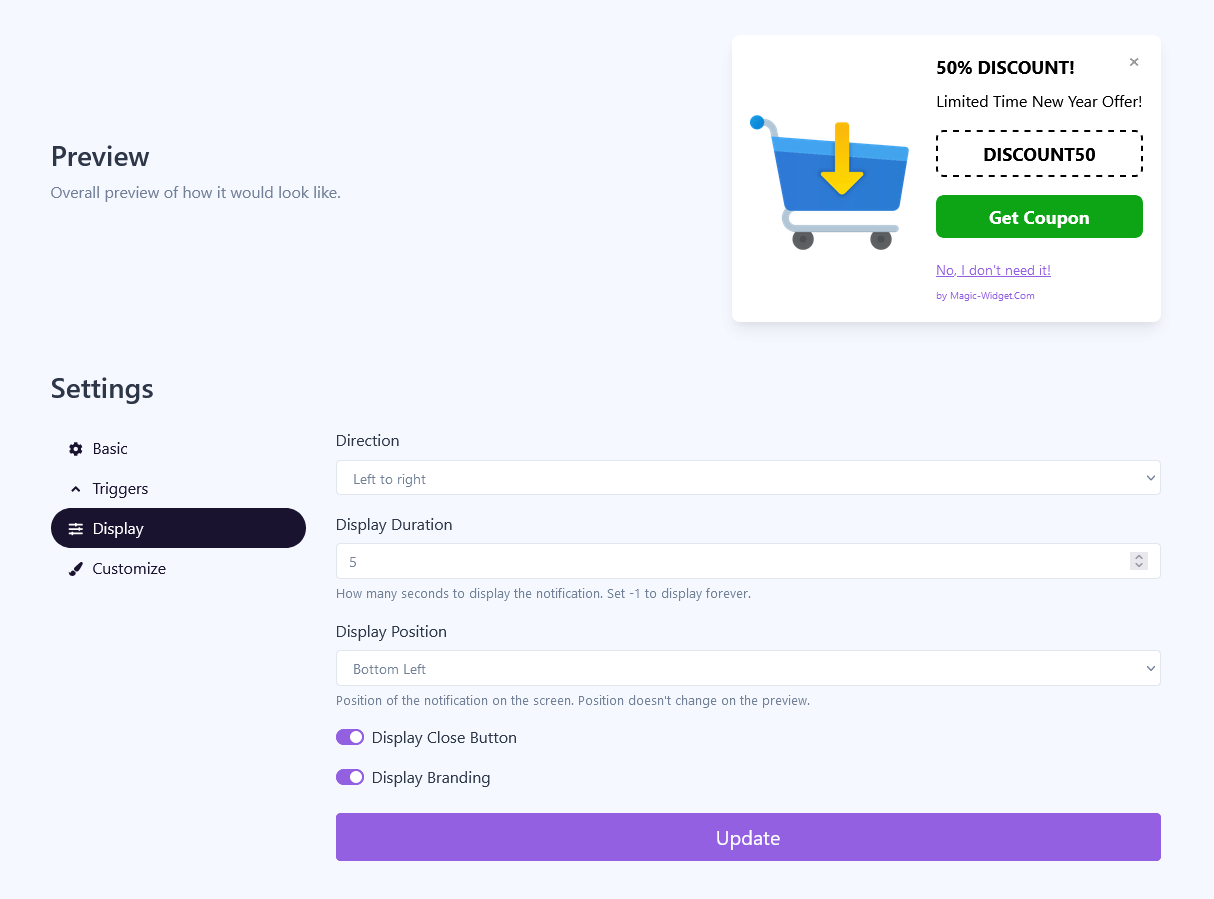This image is a screenshot of a utility settings page with a background color of an extremely light bluish-green hue. The layout suggests functionalities for configuring and previewing display advertisements.

On the left-hand side, in bold black font, the word "Preview" is prominently displayed. Directly below this, in light gray font, the descriptor "Overall preview of how it would look" provides additional context. 

At the upper-right corner of the page, there is a preview of an ad. The ad itself has a clean, white background and is square in shape. On the left side of the ad, a simple blue drawing of a shopping cart with wheels is visible, featuring a yellow arrow pointing downwards in the middle of the cart.

On the right side of the ad, bold black font announces "50% discount," followed by smaller text below that reads, "Limited time, New Year offer." Additionally, a bolded phrase "discount 50" is accentuated with a dotted line border, reminiscent of traditional newspaper coupons. Beneath this graphic, a green rectangle contains the call-to-action "GET COUPON" in white text. In smaller print below the rectangle, the option "No, I don't need it" is provided.

The lower section of the page lists various configuration options including "Direction," "Display duration," and "Display position," denoting the customizable aspects of the advertisement. At the very bottom, a long and narrow purple rectangle houses the word "UPDATE" in white text, signaling the final step to confirm any modifications made to the ad settings.